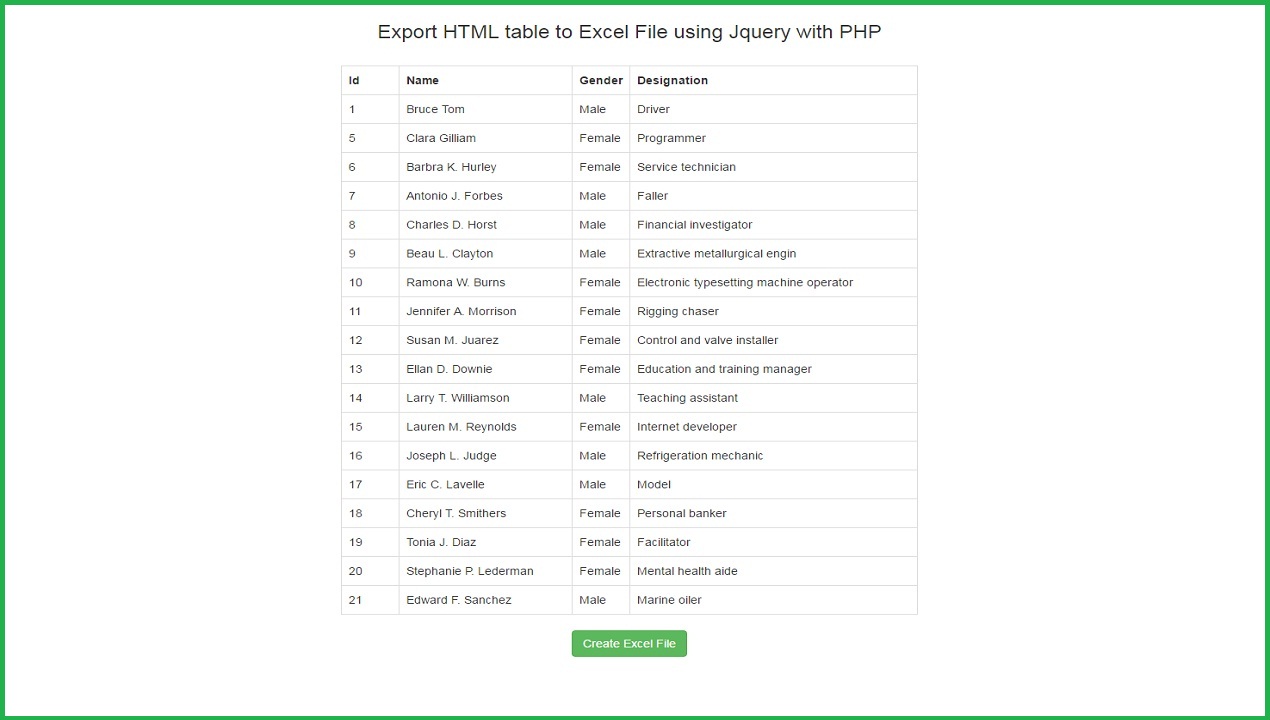The image features a green-bordered header that reads, "Export HTML Table to Excel File using jQuery with PHP." Within the image is an HTML table listing 18 rows of data. Each row includes an ID, name, gender, and occupation. Here are the detailed contents:

1. ID: 1, Name: Bruce Tom, Gender: Male, Occupation: Driver
2. ID: 5, Name: Clara Gilliam, Gender: Female, Occupation: Programmer
3. ID: 6, Name: Barbara Kate Hurley, Gender: Female, Occupation: Service Technician
4. ID: 7, Name: Tony O.J. Forbes, Gender: Male, Occupation: Father
5. ID: 8, Name: T. Horace, Gender: Male, Occupation: Financial Investigator
6. ID: P. L. Clayton, Gender: Male, Occupation: Extractive Metallurgical Engineer
7. ID: Mother 2, Appearance: But Female, Occupation: Electronic Time Setting Machine Operator
8. Name: Jennifer Morrison, Gender: Female, Occupation: Rigging Chaser
9. Name: Tuzan M. Horace, Gender: Female, Occupation: Control and File Installer
10. Name: L. N. D. Downing, Gender: Female, Occupation: Education and Training Manager
11. Name: L. R. T. Melissa, Gender: Male, Occupation: Teaching Assistant
12. Name: Lauren M. Reynolds, Gender: Female, Occupation: Underdeveloper
13. Name: Joseph O. Judge, Gender: Male, Occupation: Refrigeration Mechanic
14. Name: Eric C. Laveau, Gender: Male, Occupation: Model
15. Name: Cheryl T. Smith, Gender: Female, Occupation: Personal Banker
16. Name: Tonya J. Diaz, Gender: Female, Occupation: Facilitator
17. Name: Stephanie P. Letterman, Gender: Female, Occupation: Mental Health Aide
18. Name: Edward F. Sanchez, Gender: Male, Occupation: Marine Oiler

At the bottom of the image, there appears to be a prompt or button labeled "Create Excel File," suggesting the functionality to generate an Excel file from the displayed table data. The overall background of the image is left ambiguous.